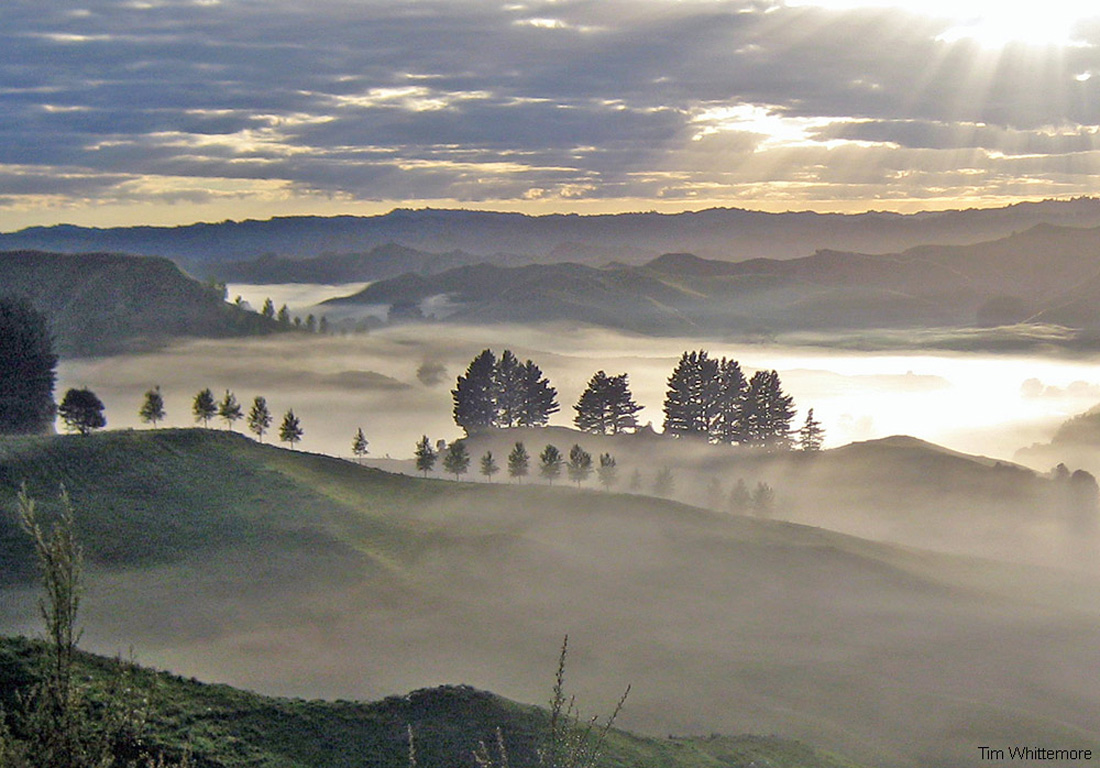A stunning landscape photograph by Tim Whitmore showcases a serene panorama of low mountains and rolling hills. The scene is enveloped in morning fog that gracefully dips into the valleys, while the Sun breaks through a partially overcast sky in the top right corner, casting a brilliant light. The foreground features a green cliff edge with a few scattered weeds in the lower left-hand corner. The mist clings to the grey hills, creating a magical atmosphere as rows of pine trees stand along the first hills, with larger trees dotting the subsequent hillsides. Further in the distance, the fog, possibly tule fog, blankets what might be water—suggesting an ocean or lake—before another series of mountains rise up. The horizon is lined with layers of dark clouds interspersed with beams of sunlight. Amidst the lush greenery and undulating terrain, the diverse foliage—from vibrant greens to earthy browns—adds to the richness of the scene. The photograph is signed in the bottom right corner by the photographer, Tim Whitmore.